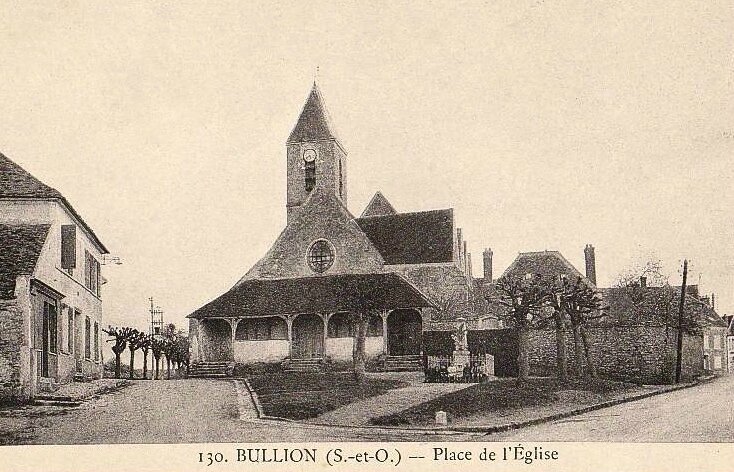This grainy black and white photo, evocative of early 20th-century photography, captures an old church prominently titled "130 Bullion, Place de l'Anglais" at the bottom. The church, centered in the image, features a steep black roof and a tall steeple with a clock. A distinctive oval stained glass window adorns the front, beneath a triangular roof. The spacious porch, encircled by white fencing, offers three arched entryways. The surroundings include manicured grass, trees, and a cement monument in the churchyard.

Positioned at a Y intersection, the church is flanked by a building with shutters on one side and residential homes with a telephone pole on the other. The left side of the scene showcases a white building and a clear view of several palm trees at the road's end. A concrete sidewalk and pathway lead to the entrance, contributing to the historical charm of this picturesque, grainy snapshot.